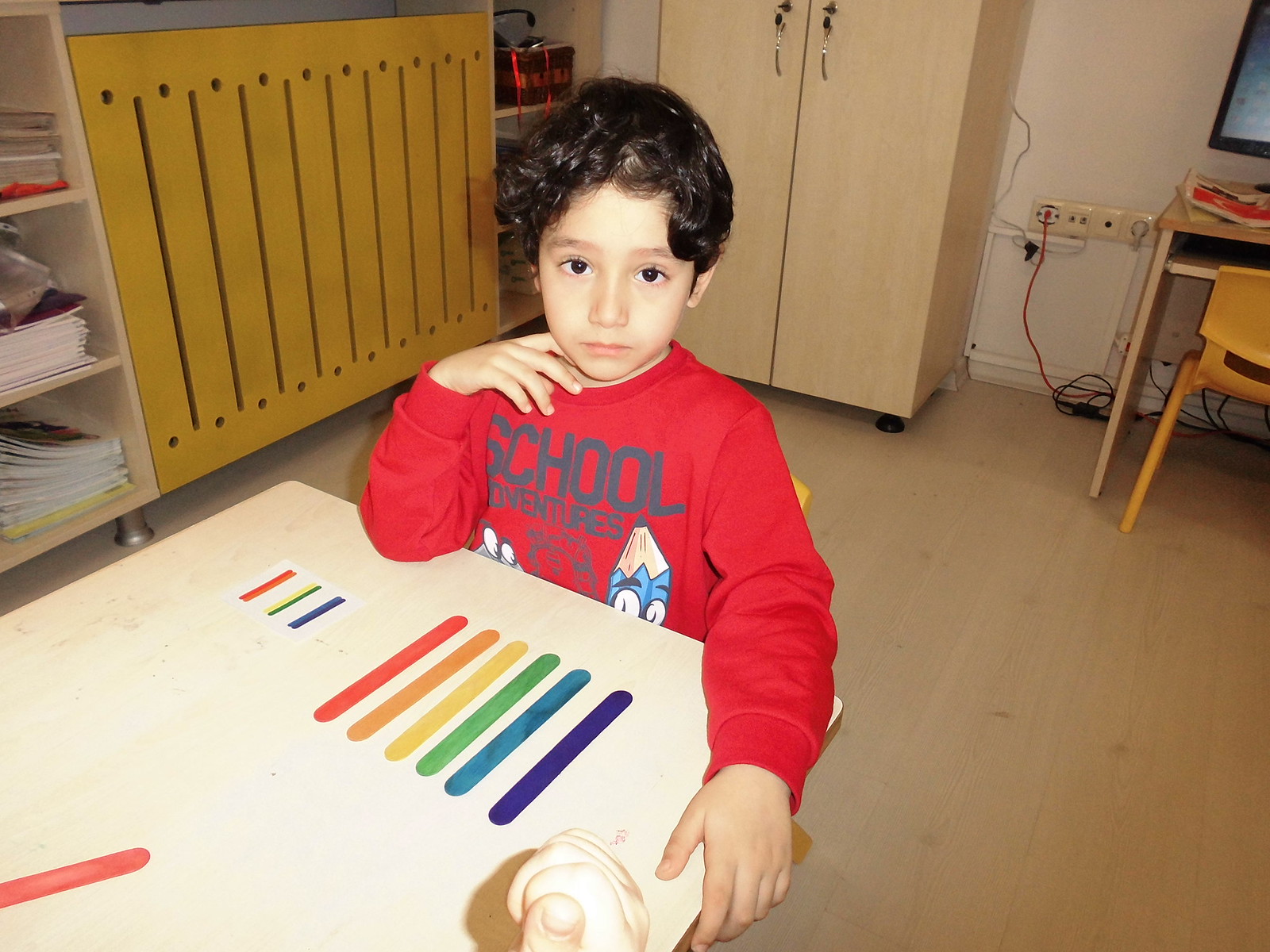In the image, a young boy, appearing to be around six years old, is seated at a small white table. The boy, with short, curly black hair, is wearing a red long-sleeve shirt adorned with a blue pencil illustration and the text "School Adventures." He is positioned on a child-sized yellow chair and looks directly at the camera. Spread out in front of him on the table are multicolored popsicle sticks—red, orange, yellow, green, blue, indigo, and a pale blue stick—suggesting a craft or educational activity.

The setting resembles a classroom, characterized by various educational tools and furniture. In the background, a small wooden desk with a computer monitor is situated along with another yellow chair. Above this desk, shelves display an array of notebooks and magazines. Additional elements in the background include a white cabinet, a brown closet with silver handles, and a red lunchbox. The light brown, wooden floor adds warmth to the environment, while visible outlets and cords, including a red cord plugged into one outlet, add practical details. A glimpse of another hand is noticeable at the bottom of the frame, suggesting the presence of another person nearby.